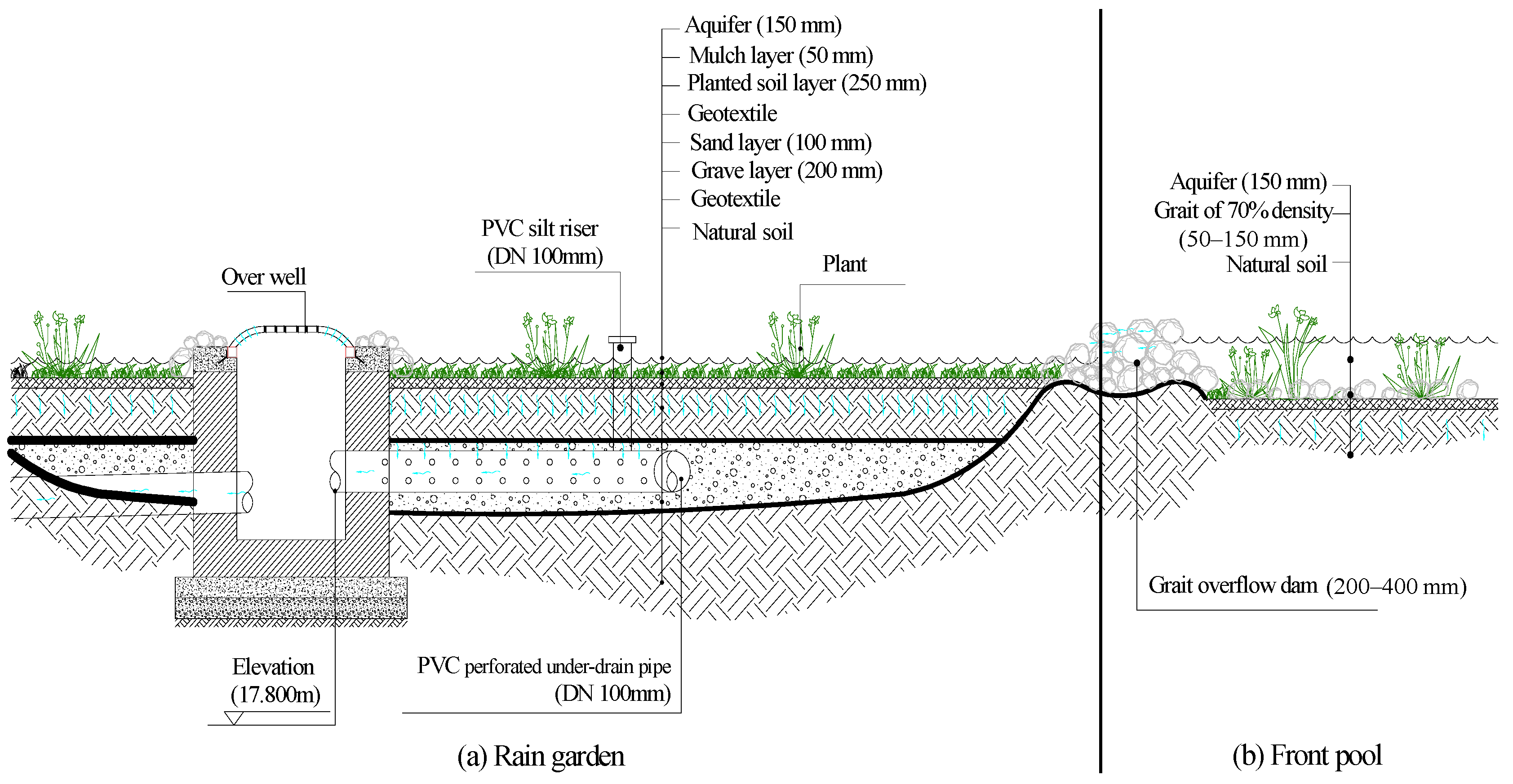This detailed color illustration, likely from a book or pamphlet, provides a comprehensive cross-section of an underground landscaping design, emphasizing the functionality and layout of a rain garden and associated water management features. 

At the top layer of the diagram, green grass and shrubs are depicted, showcasing a typical garden surface. Below this surface, various underground structures and materials are meticulously detailed. Starting from the left, a rectangular section labeled "over well" indicates an elevation of 17.800 meters. This section is connected to a PVC silt riser (DN 100 millimeters) and further down to a PVC perforated underdrain pipe (DN 100 millimeters), which is an integral part of the rain garden system.

Central to the diagram are distinct layers of soil and materials, each with a specific function. These include:
- Aquifer
- Mulch layer
- Planted soil layer
- Geotextile layer
- Sand layer
- Gravel layer
- Another geotextile layer
- Natural soil

These layers are vital for the proper filtration and management of rainwater to prevent over-saturation and flooding. The illustration also includes a depiction of a plant rooted in these soil layers, symbolizing the garden's vegetation.

To the right side of the diagram, additional labels and structures are present, such as another mention of the aquifer, a grate with 70% density, and natural soil. At the bottom right, the front pool is highlighted, illustrating the final destination for excess water managed by this system.

Overall, this diagram serves as a detailed reference for understanding the construction and layers involved in creating a sustainable and efficient rain garden, ensuring proper drainage, water management, and plant health.